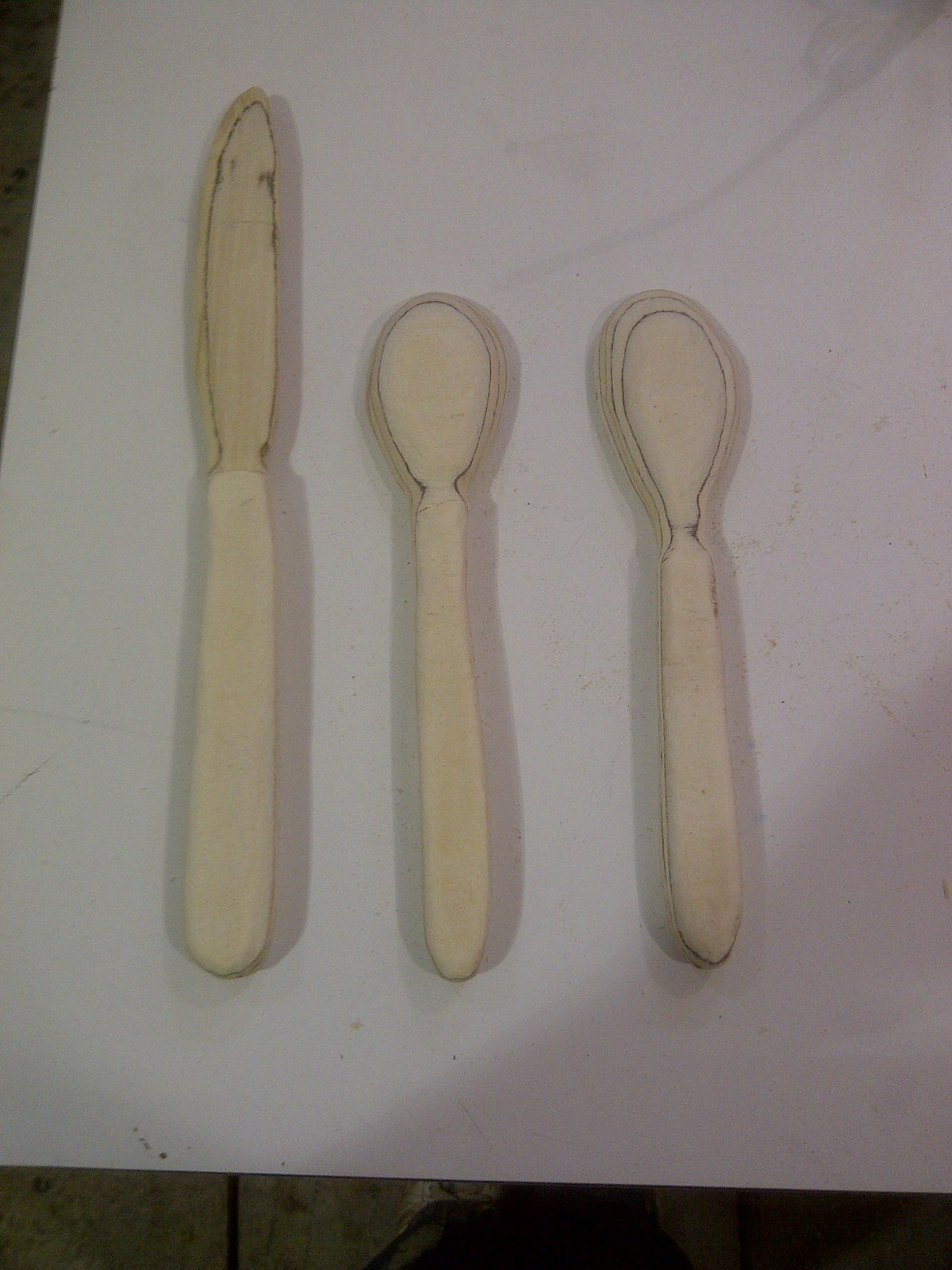The image showcases three beige, manila-colored utensils—which appear to be made of wood or plastic—arranged on a white surface. From left to right, the items are a butter knife, followed by two spoons of slightly different shapes. The knife has a distinctive black line reminiscent of rust along its blade, and possibly some mold growing on its tip. The spoons have irregular, slightly oval-shaped heads with black lines drawn along their edges and handles, adding a crafted or decorative element to their appearance. Although the utensils look functional, they appear more like molded plastic imitations or decorative pieces rather than practical tools for eating, given their jagged and imperfect shapes. The image extends down to reveal a section of very dirty, dark grayish-green tiled flooring beneath the white surface.